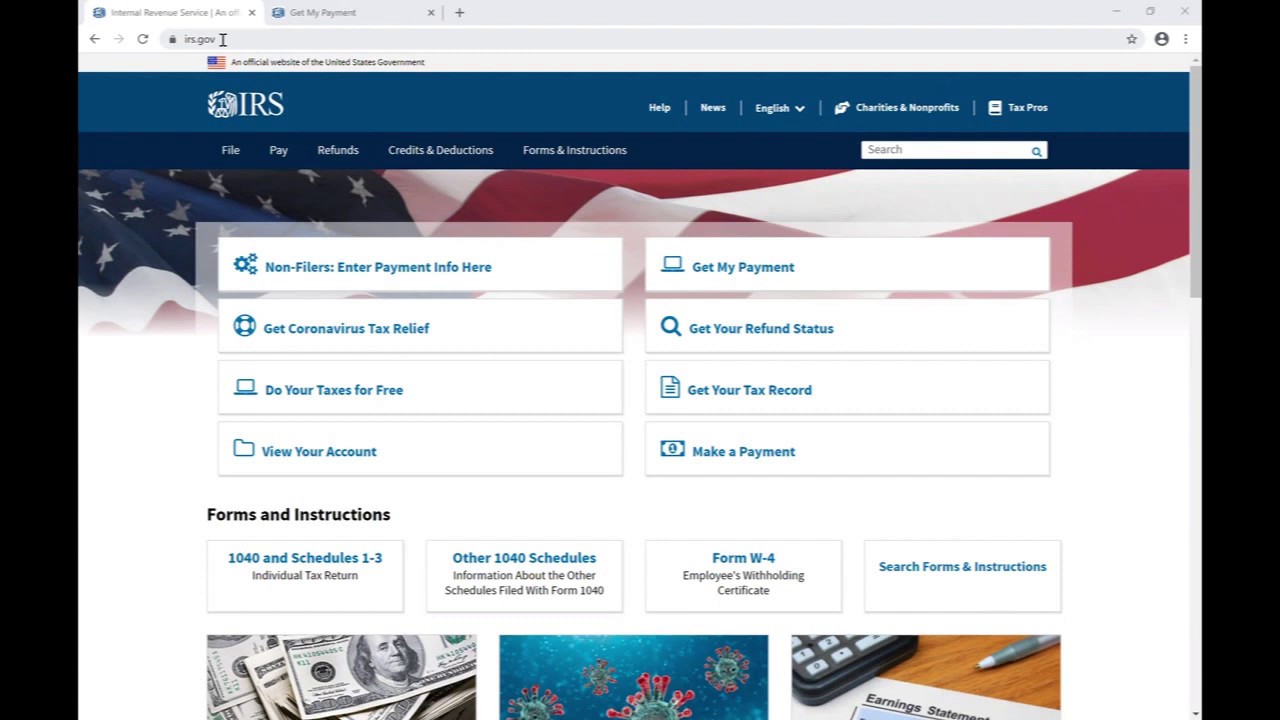The image depicts the official IRS website, IRS.gov, open on a web browser, possibly Microsoft Edge or another browser. The webpage features an elegant background with an American flag. At the top of the page, there are two open tabs: one for "IRS Services" and another for "Get My Payment."

At the forefront, a prominent blue tab displays the word “IRS,” flanked to the right by a menu with options such as Help, News, English, Charities & Nonprofits, and Tax Pros. Below this, a darker blue navigation bar provides quick access to essential categories: File, Pay, Refunds, Credits and Deductions, and Forms and Instructions. A search bar is positioned beneath this navigation panel.

The main section of the page showcases a diverse selection of white buttons against the backdrop, offering services including "Enter Payment Information Here," "Get My Payment," "Get Coronavirus Tax Relief," "Get Your Refund Status," "Do Your Taxes for Free," "Get Your Tax Record," "View Your Account," and "Make a Payment."

Further down, there are detailed links for Forms and Instructions such as 1040 and Schedules 1 through 3, Individual Tax Return, other 1040 schedules, information on scheduling and filing with Form 1040, Form W-4 (Employee's Withholding Certificate), and a search function for forms and instructions.

Complementing the informational text, the page also features several relevant images, including icons of a virus, $100 bills, and an Earnings Statement, providing a visual context to the offered services.